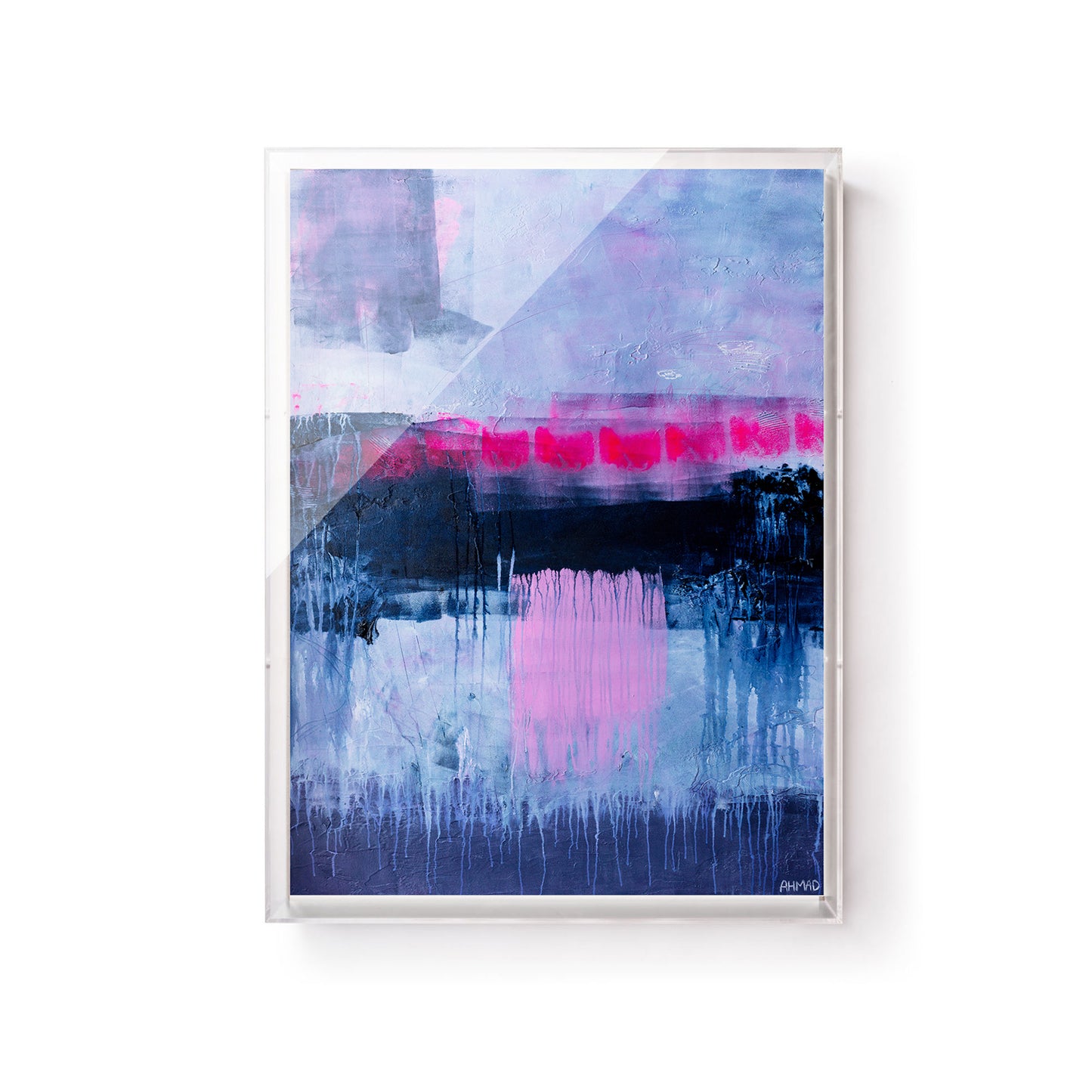This is an abstract painting showcased on a white or clear-framed piece of paper. The artwork, signed by Ahmaud at the bottom right, features a harmonious blend of pastel colors with a predominant theme of blue and pink. The top half of the painting consists of lighter pastel blues and pinks, with sections where dark pink splotches, resembling hot pink, are interspersed. Below this, a prominent, horizontal navy blue section divides the painting, which adds depth and contrast. Below the dark blue stripe, the paint appears to have been allowed to drip and streak downwards, mimicking the effect of watercolor with excess water, creating vertical lines in varying shades of blue. Interspersed within these drips are defined vertical strokes of pink, adding structure amidst the flowing lines. Overall, the painting evokes a sense of fluidity and melting colors, masterfully blending darker and lighter hues to create a captivating visual experience against a background that appears to be white.